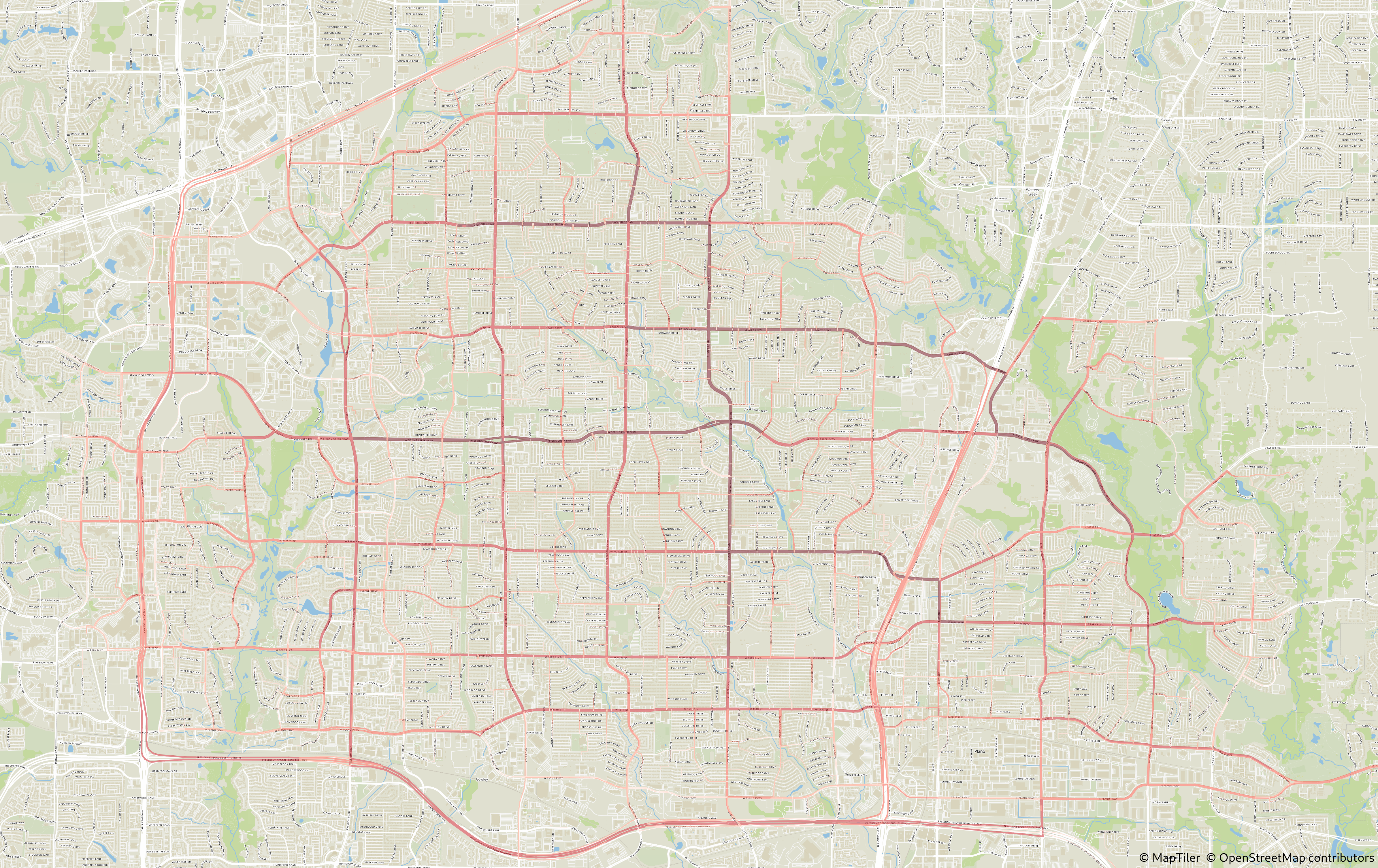This image features a detailed map with indistinct text due to its small font size, making it difficult to determine the specific location it represents. In the bottom right corner, the map is credited to "Map Tyler, OpenStreetMap Contributors." The primary color scheme of the map is a very light beige background, which is overlaid with various lines in multiple colors and thicknesses to denote different features. 

Green areas are likely representing parks or forests, while blue areas denote bodies of water such as lakes and rivers. The white lines on the map seem to highlight major roads and highways, providing an important guide to the transportation networks in the area. Meanwhile, red lines are prominently featured in the central part of the map, forming an irregular, almost square-like pattern, with some lines appearing darker than others, possibly indicating roads or boundaries of higher significance. The overall visual layout presents a complex and detailed cartographic representation of the unknown location.